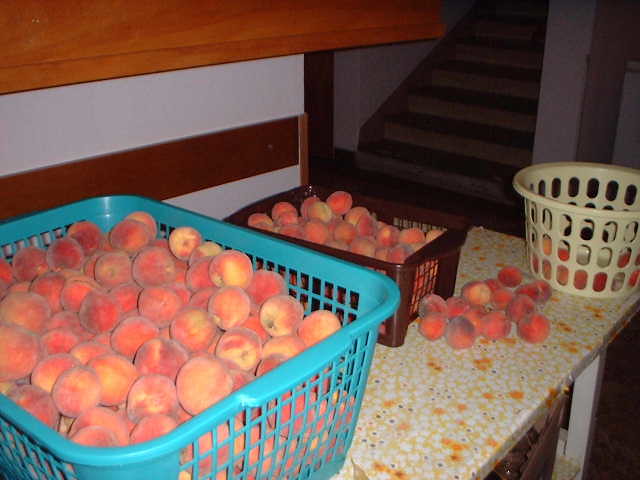The color photograph displays three plastic crates filled with ripe, variegated peaches in shades of orange and yellow. On the left, an aquamarine rectangular basket brims with approximately a hundred peaches. To the right, a smaller brown square basket is similarly filled with peaches, while between them sits an off-white, beige, rounded laundry-type basket, also loaded with peaches. All three containers rest atop a light beige kitchen worktop speckled with orange circles, suggesting either a patterned design or splatters of peach juice and fruit flesh. The background reveals a staircase with dark risers and light footpads, ascending into shadows, flanked by white walls with honey-colored wooden accents. Several loose peaches are scattered on the counter, adding to the abundance. The scene is set within a dimly lit home, with the kitchen and staircase subtly illuminated.